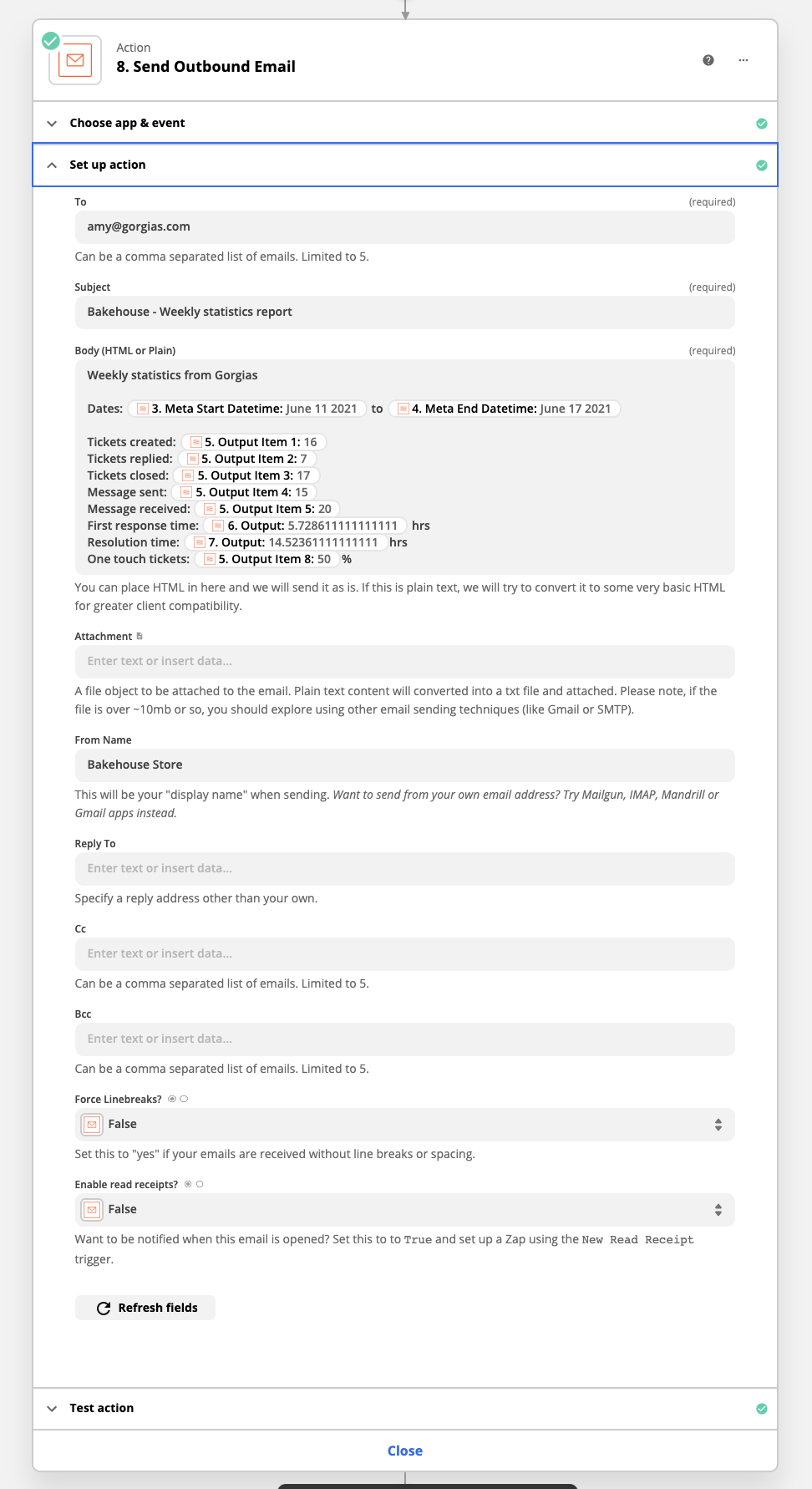This image shows an email automation setup interface. At the top, there is a header indicating the action: "B Send Outbound Email." Below this, there is an icon featuring a small box with a piece of mail and a green checkmark. The next section has the label "Choose App and Event" with a downward-pointing arrow. On the right side of this section is a green circle.

Further down, the interface shows another section labeled "Set up Action" with an upward-pointing arrow on the far right, also accompanied by a green circle. This area contains multiple text fields and settings. 

- The recipient's email field is filled out with "to: Amy@Georgia.com," noting that it can be a comma-separated list limited to five addresses.
- The subject line is "Bakehouse Weekly Statistic Report."
- The body section allows for HTML or plain text and contains language like "Weekly status from Georgia dates" and other statistical data.
- There are metrics labeled "tickets created" followed by numbers, although the text is small and difficult to read.
- All text is presented in black on a white background.

Additional settings include:
- A section for attachments with a label "From Name: Bakehouse Store."
- A field labeled "Reply-To" with an input box.
- Options marked as "False" for certain settings.

At the bottom, there is a "Refresh Fields" button, followed by a selection bar with the options "Test Action" and "Close" located at the center of the bottom bar.

The background of the entire interface is white, providing a clean and organized layout.